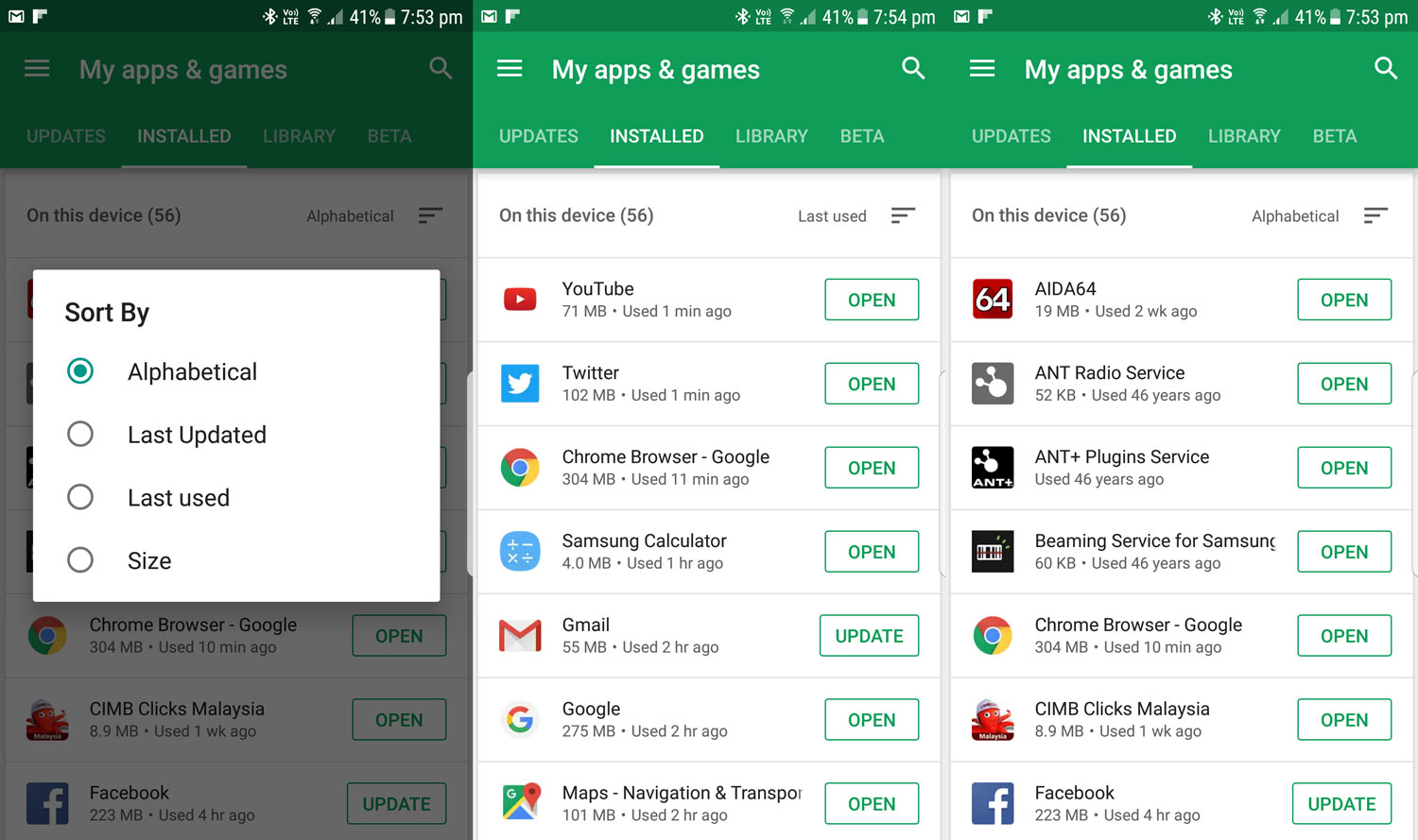Here is a cleaned-up and detailed caption for the series of images:

"The series of images, shown side-by-side, depicts navigation through an Android device's 'My Apps & Games' section. The sequence starts with the user viewing their installed apps sorted by usage, where YouTube and Twitter, both used within a minute, are listed at the top. In the second image (chronologically first), a white pop-up titled 'Sort By' appears, offering sorting options. The user selects 'Alphabetical' from the dropdown menu. The final image displays the apps reorganized alphabetically, confirming the new sorting order. Each image features the familiar green banner at the top, allowing navigation through updates, installed apps, the library, or beta programs."